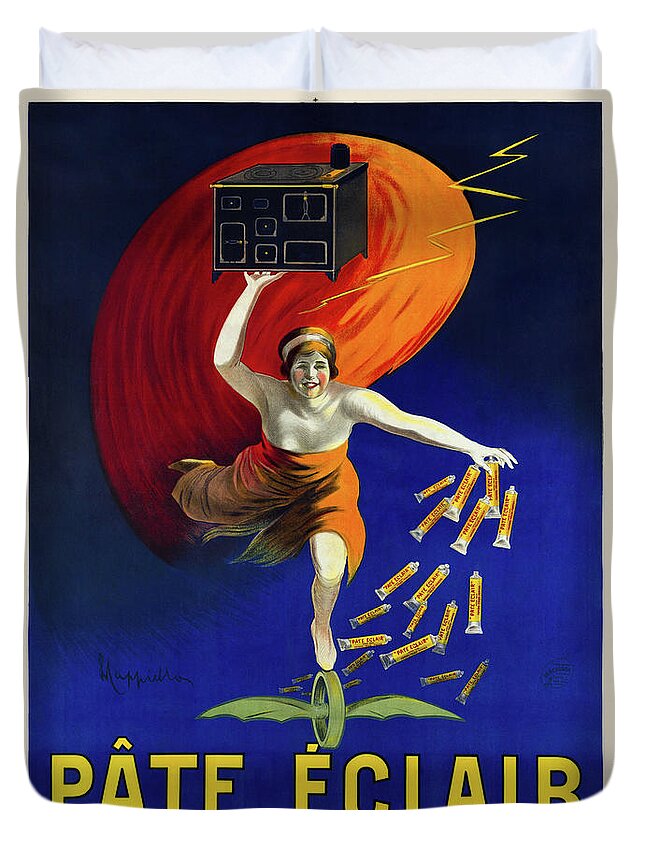This is a vibrant, visually arresting image that appears to be the cover of a book or an old-timey French advertisement. Dominated by rich, dark blue hues that transition to lighter blue towards the bottom, the image is centered around an intriguing female figure. She is dressed in a sleeveless, orange dress that falls to her knees and has matching orange hair. 

The woman is balanced delicately on one foot atop a wheel, which intriguingly, sports bat-like wings. Her right leg is kicked back, adding a sense of dynamic motion to the scene. In her right hand, extended overhead, she holds what looks like a small black storage cabinet or stove. 

Behind her is a striking large orange circle that contrasts sharply with the dark blue background. This circle is complemented by a lightning bolt that ascends towards the upper right corner, adding an element of energy and drama to the composition.

Her left hand is outstretched, releasing a cascade of yellow tubes that resemble paint or possibly toothpaste, all labeled "Pate Eclair." The words "Pate Eclair" are also prominently displayed in yellow at the bottom of the image, although part of the text is partially obscured. Above this text is an indistinct signature that appears to read "Mapolillian."

Overall, this detailed artwork offers a whimsical yet dramatic portrayal infused with rich colors and fantastical elements.